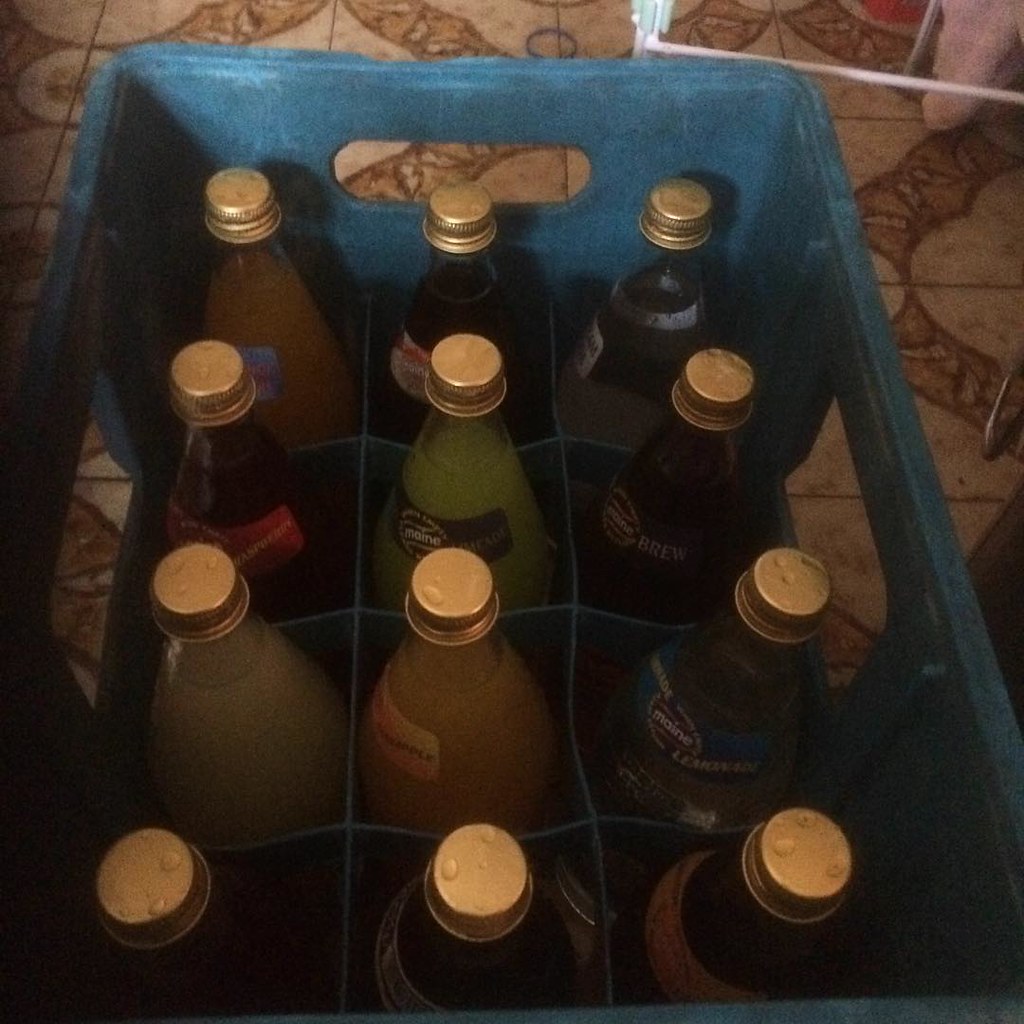A slightly top-down but angled view captures a teal plastic crate, arranged vertically, containing 12 glass bottles with plain gold caps. The crate, with handles on all four sides, rests on a hard, light-tan flooring that seems to be made of a non-wood material and features a circular design pattern. The bottles inside are uniform in shape, being short and stout, holding various colored liquids ranging from clear, yellow, green, and multiple darker hues. Many of the bottles have labels with "Maine" written in lowercase white letters. The natural light spilling from a nearby window suggests the photo was taken indoors, likely near a window.